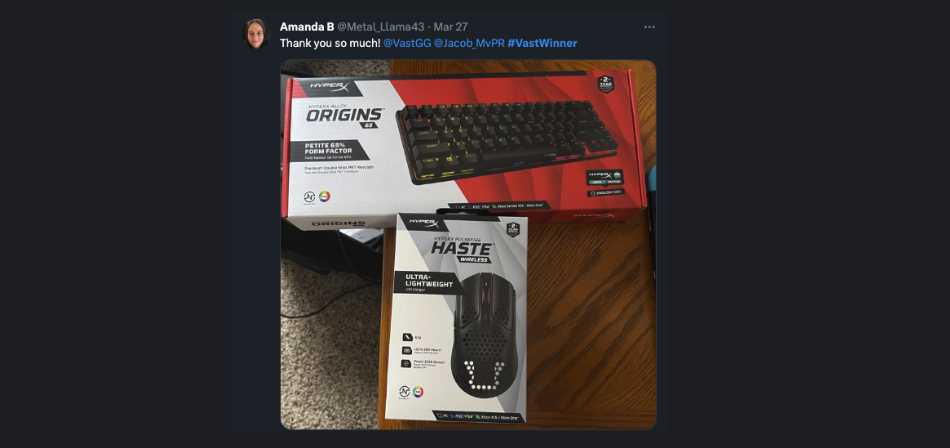Screenshot of a Post from Amanda B's Facebook Page

In the image, a Facebook post is prominently displayed against a black background. At the center of the post is Amanda B's profile picture, showing her smiling face. Dated March 27th, the post expresses gratitude, reading: "Thank you so much @vast_GG @Jacob_MVPR #vastwinner".

Amanda B has tagged @metal_llama43 in her post, which showcases a photo of a computer keyboard and mouse. The products are still in their boxes, placed on a brown table. The table stands on a tan carpet, visible below. The first box, housing the keyboard, is a white and red rectangular package labeled "Origins 44," with the black keyboard visible inside. Next to it, the white box containing the black mouse is marked "Haste Ultra Lightweight," along with additional product information.